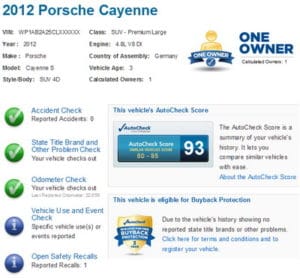This detailed image captures a screen displaying comprehensive information about a 2012 Porsche Cayenne. The layout consists of multiple organized sections. On the left, five distinct areas provide various details about the vehicle. Meanwhile, to the immediate right of this section, another column with five more distinct areas continues down the middle of the screen.

Significant focus is given to the vehicle’s ownership history. Positioned towards the right portion of the image is a highlighted section marked "One Owner" beside a checkmark icon; this area is accented with a distinctive blue-green color. Accompanying this, a small silhouette of a person is positioned above or below the "One Owner" banner, reinforcing the vehicle's single ownership status.

Below this ownership section on the left are five circular icons. The top three circles are green, each adorned with a white checkmark, indicating successfully cleared checks for "Accident Check," "State Title Brand and Other Problem Check," and "Odometer Check." The bottom two circles are blue with lowercase letter 'i' icons, indicating pending checks for "Vehicle Use and Event Check" and "Open Safety Recalls." This comprehensive visual profile delivers an in-depth overview of the vehicle's history and condition.